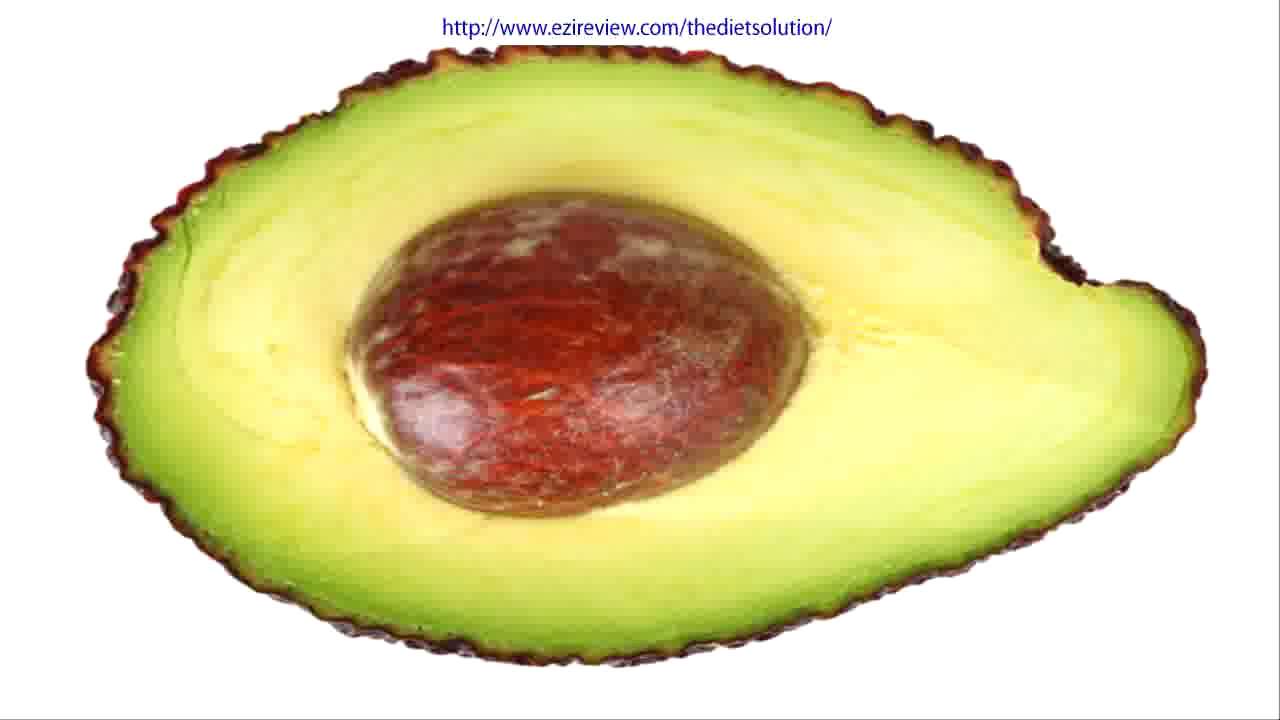The digital photograph captures a close-up view of a neatly sliced avocado, revealing both halves prominently displayed against a completely white background. The texture of the avocado's flesh is evident; it is a bright green color that fades to almost light yellow near the center, where the large, oval pit resides. The pit itself is a reddish-maroonish brown, nestled within the creamy green flesh. Notably, the outer skin of the avocado is shown in realistic detail, boasting a lumpy, wrinkly, and jagged texture rather than a smooth exterior, which is commonly depicted in illustrations. The green edge of the flesh touches the thin outer brown skin. Floating just above the avocado image is blue text that reads "http://www.eziereview.com The Diet Solution", providing an additional contextual layer to the visual.